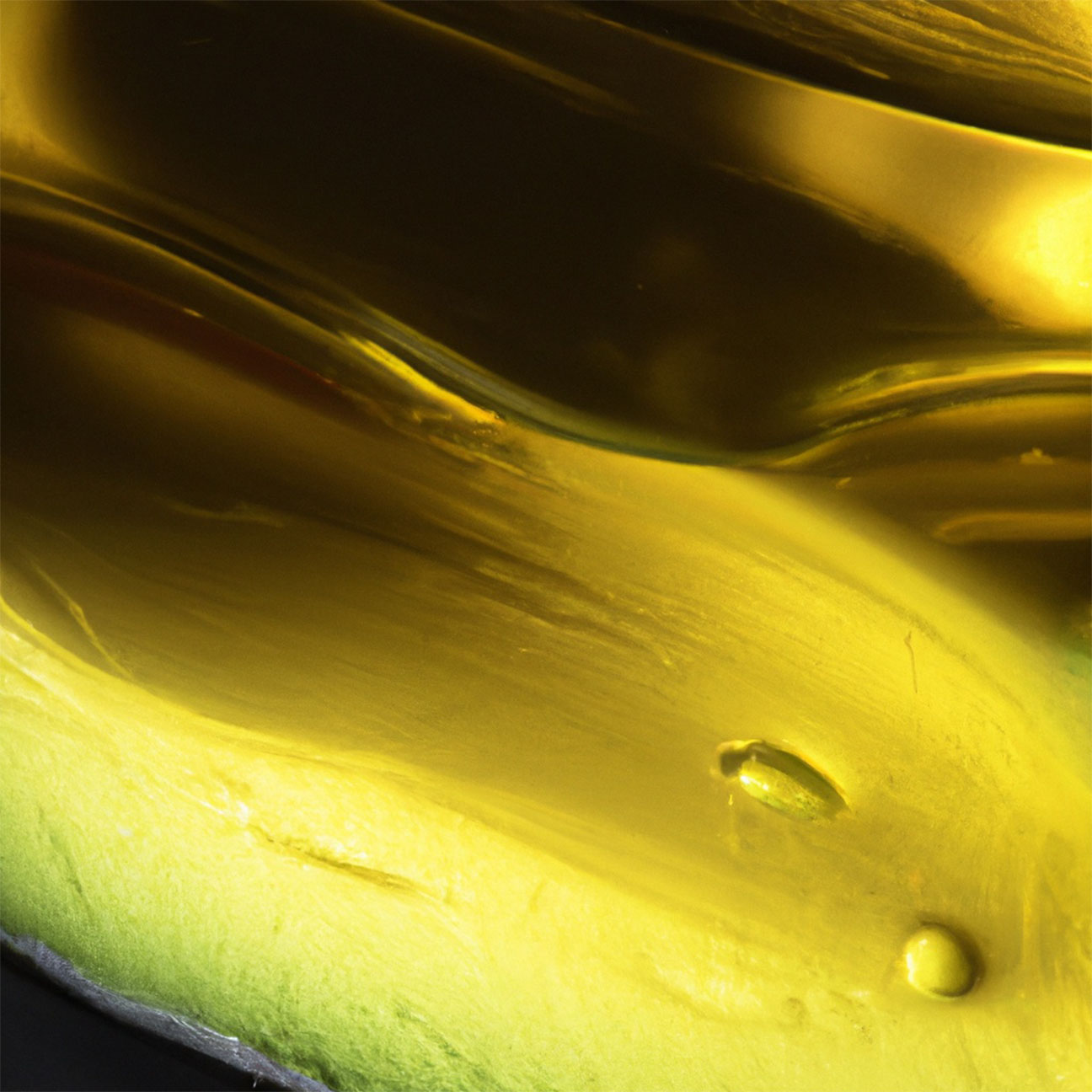This photograph appears to be a highly detailed close-up image that resembles the interior of an avocado but could also be interpreted as something else due to the visual details presented. The bottom part of the image exhibits a dark grayish color, akin to the exterior skin of an avocado. Right above this, there's a vivid layer of bright green, reminiscent of the avocado flesh just beneath its peel. Moving further into the image, the predominant area is a smooth, creamy yellow shade typical of an avocado's inner texture. However, the image has characteristics that suggest it might be something different. The golden color and small bubbles within this gold area hint at the possibility of it being gold paint, possibly magnified, showcasing a textural and color shift that includes green hues and a small silver sliver at the corner. The structure of the image undulates like a hill range, with the top portion featuring an indentation transitioning into a black color, possibly indicating a liquid surface or paint that has oxidized.